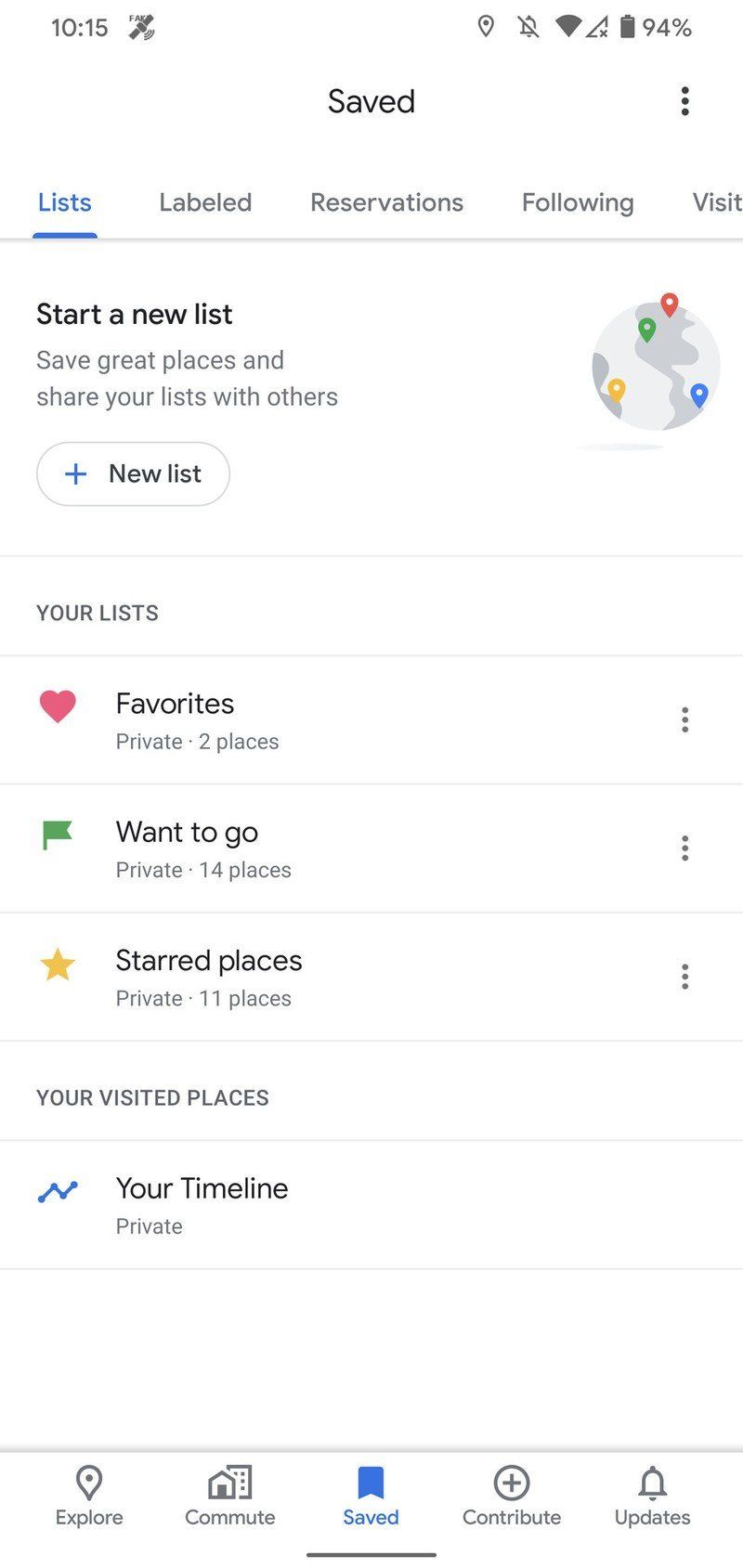A detailed caption for the image described might look like this:

---

The image displays a smartphone screen with a white background. At the top left, the time is shown as 10:15. On the right, the battery icon indicates 94% charge, and notifications are silenced. There is a location icon and several other unidentified icons along the top. 

Below this status bar, "Saved" appears in black text centered on the screen, with three vertical dots for additional options on the far right. Directly beneath this are five selectable options in a horizontal row: Lists, Labeled, Reservations, Following, and Visited. The "Lists" option is highlighted in bright blue text with a corresponding underline, while the remaining options appear in gray. 

A light gray line separates these options from the content below. In the main section, the prompt "Start a new list" appears in black text, with the subtext "Save great places and share your lists with others" in gray below it. A button labeled "New List" in black text with a bright blue plus sign is positioned alongside a globe graphic in light and dark gray, adorned with colorful location pins in red, blue, yellow, and green.

Below this section, a pale gray line delineates the space. The heading "YOUR LISTS" appears in gray, all caps text followed by another faint gray line. The "Favorites" section is next, marked by a black text label with a red heart icon to the left; under it, the text "Private - 2 places" is in gray. Another faint gray line leads to "Want to Go" in black text, which is labeled "Private - 14 places" in gray, accompanied by a green flag icon. Following another faint gray line, "Starred places" is listed in black text with a gold star icon; beneath it, "Private - 11 places" is noted in gray.

Further down, another faint gray line introduces the "YOUR VISITED PLACES" section in gray, all caps text, followed by "Your Timeline" in black text. The associated subtext "Private" is displayed in gray beneath it, concluding the screen's content.

---